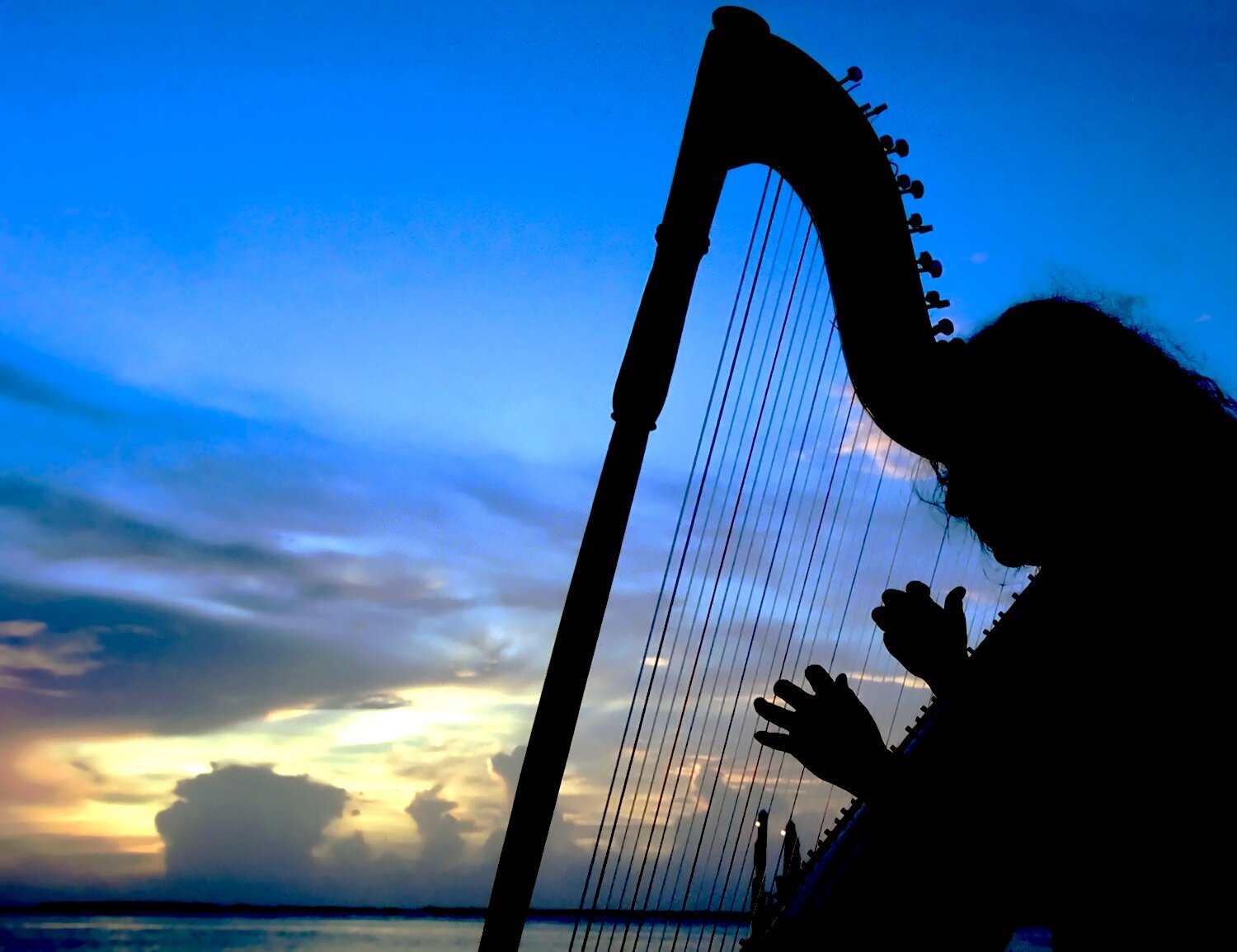In this captivating photograph, a lady is poised to play a harp by the ocean at sunset. The scene is awash in a spectrum of colors, with a striking blue sky that dominates the upper half of the image, gradually fading into vibrant oranges and yellows as the sun begins to set. The bottom of the sky is dotted with blue clouds streaking across the horizon. The woman's silhouette, characterized by her long, dark hair and graceful posture, is perfectly framed against the glowing backdrop. Her fingers rest delicately on the strings of the harp, which leans into her, capturing every individual tuning peg in crisp detail. The image also features two mysterious upright structures with lights emanating from them in the background, adding an element of intrigue to the serene coastal setting.